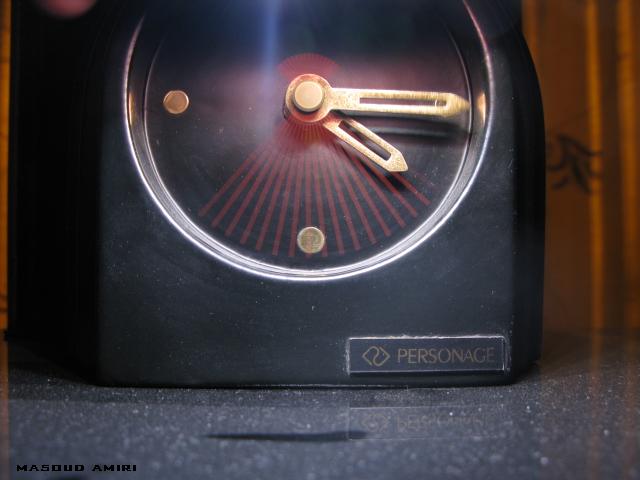This detailed image captures a close-up of a modern desk clock, likely used as a baking timer, with a clear focus on its distinctive features. The clock has a black, smooth surface with a dust-speckled top, interrupted by a darker line suggesting someone ran a finger through the dust. Its base is flat, with sides that rise straight up and curve into a dome at the top. The clock face is round and black, covered by a circular glass pane revealing its intricate interior.

Prominently, the clock features two large, silver hands; one points to the top right, while the other angles to the bottom right. Gold knobs mark the 3, 6, 9, and 12-hour positions, complemented by two gold dots at the 6 and 9 positions. Radial lines extend from the center in a fan shape, purely decorative. The inside also includes visible screws on the left and bottom center.

A small, rectangular plaque in the bottom center of the clock face displays the brand name, which is somewhat obscured but reads "Personage" or "Personance." The background features a yellow curtain, giving a warm, indoor ambiance to the setting. Overall, this clock combines practical design with decorative elements, making it a visually appealing and functional piece.